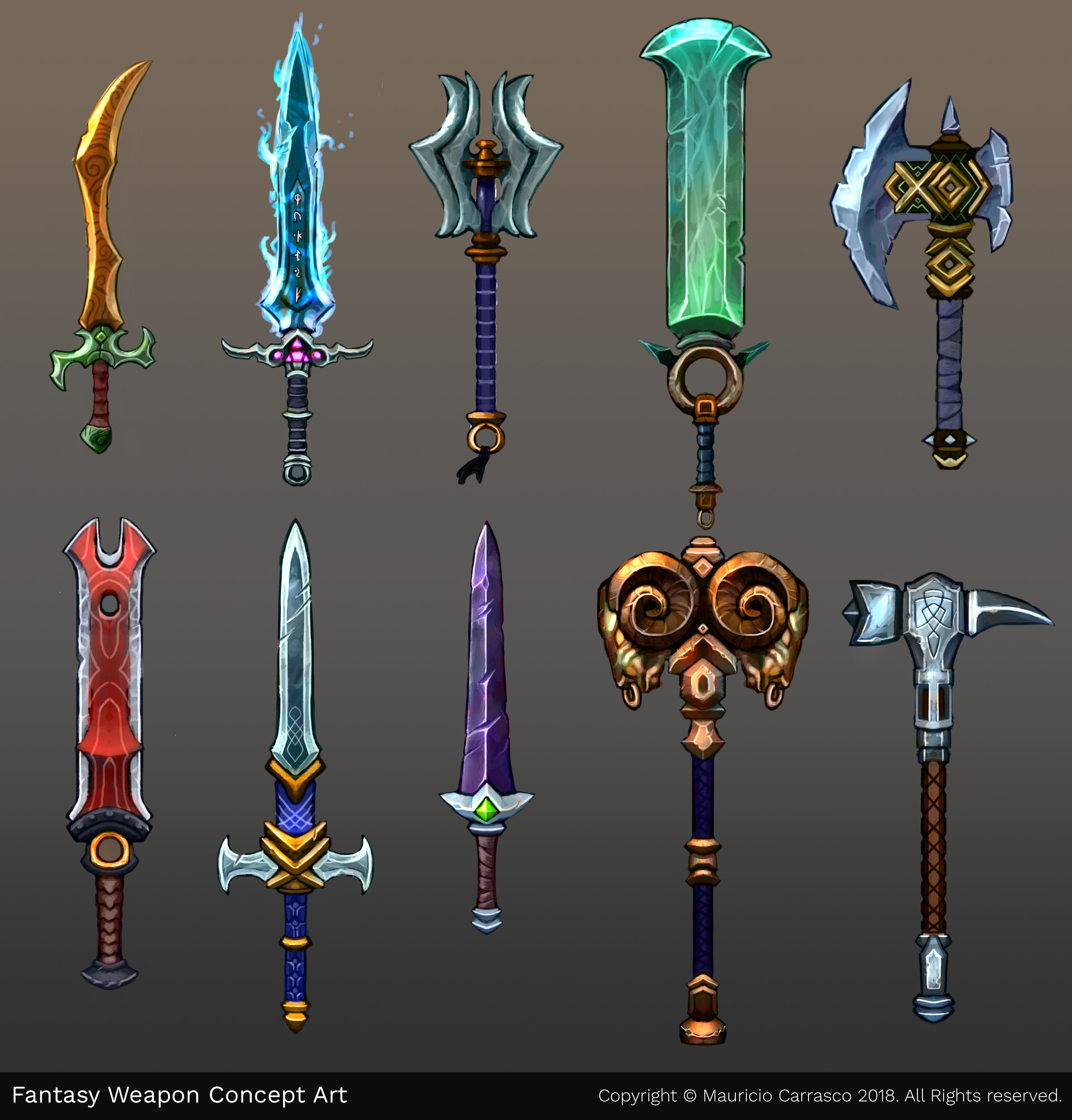This image features a collection of ten uniquely designed, computer-generated fantasy weapons, arranged in two rows of five against a dark gray and light gray background. The caption at the bottom of the image reads, "Fantasy Weapon Concept Art," with the credit "Copyright C. Mauricio Carrasco, 2018. All Rights Reserved."

The weapons, depicted in a vibrant and cartoonish fantasy style, showcase an array of swords, axes, hammers, and other martial implements. Each weapon boasts its own distinct shape and coloration, with brilliant hues including purple, blue, red, green, gold, silver, and bronze.

In the top row, from left to right:
1. A gold scimitar with a green handle.
2. A glowing blue sword inscribed with runes and adorned with a silver handle and a purple jewel.
3. A purple-handled weapon with golden elements and silver wings encircling it.
4. A wide, seafoam green sword with a circular handle, appearing to be made of jade.
5. A tribal-style hatchet with a blue blade, gold detailing, and a gray handle.

In the bottom row, from left to right:
1. A red and silver sword with a wide blade, notched edges, and a hole in the middle.
2. A traditional-looking blue sword with silver accents.
3. A simple sword featuring a dark violet blade with a silver and brown hilt.
4. A large war hammer, ornamented with back-to-back ram’s heads.
5. Another hammer, designed with a Celtic-inspired emblem on its steel head and a brown handle.
  
The detailed and imaginative design of the weapons, combined with their striking colors and intricate shapes, make this concept art an eye-catching piece likely intended for a sci-fi or fantasy game or media property.